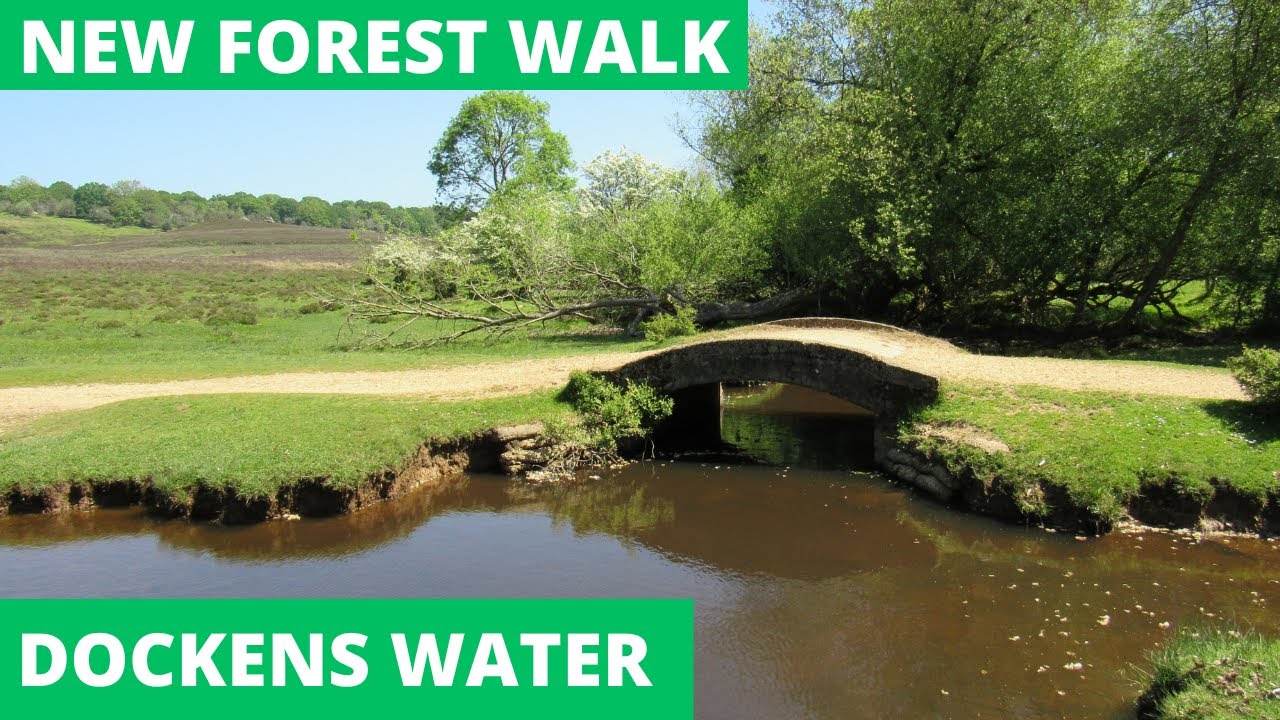The image is an advertisement for a scenic pathway, titled "New Forest Walk," which is prominently displayed in bold white text on a green banner in the top left corner. Additionally, the text "Dockins Water" is situated on the bottom left. The central focus is a serene pond with a bridge spanning its narrow width, accompanied by a dirt path that meanders through the middle. The background in the top right features a cluster of trees providing a lush canopy, while the top left reveals a clear blue sky over an open field, capturing the essence of a warm summer day. The dirt path is bordered by a combination of grassy patches and floating leaves in the pond, particularly noticeable in the bottom right corner. The image projects a well-lit, inviting scene, ideal for a peaceful walk through nature.